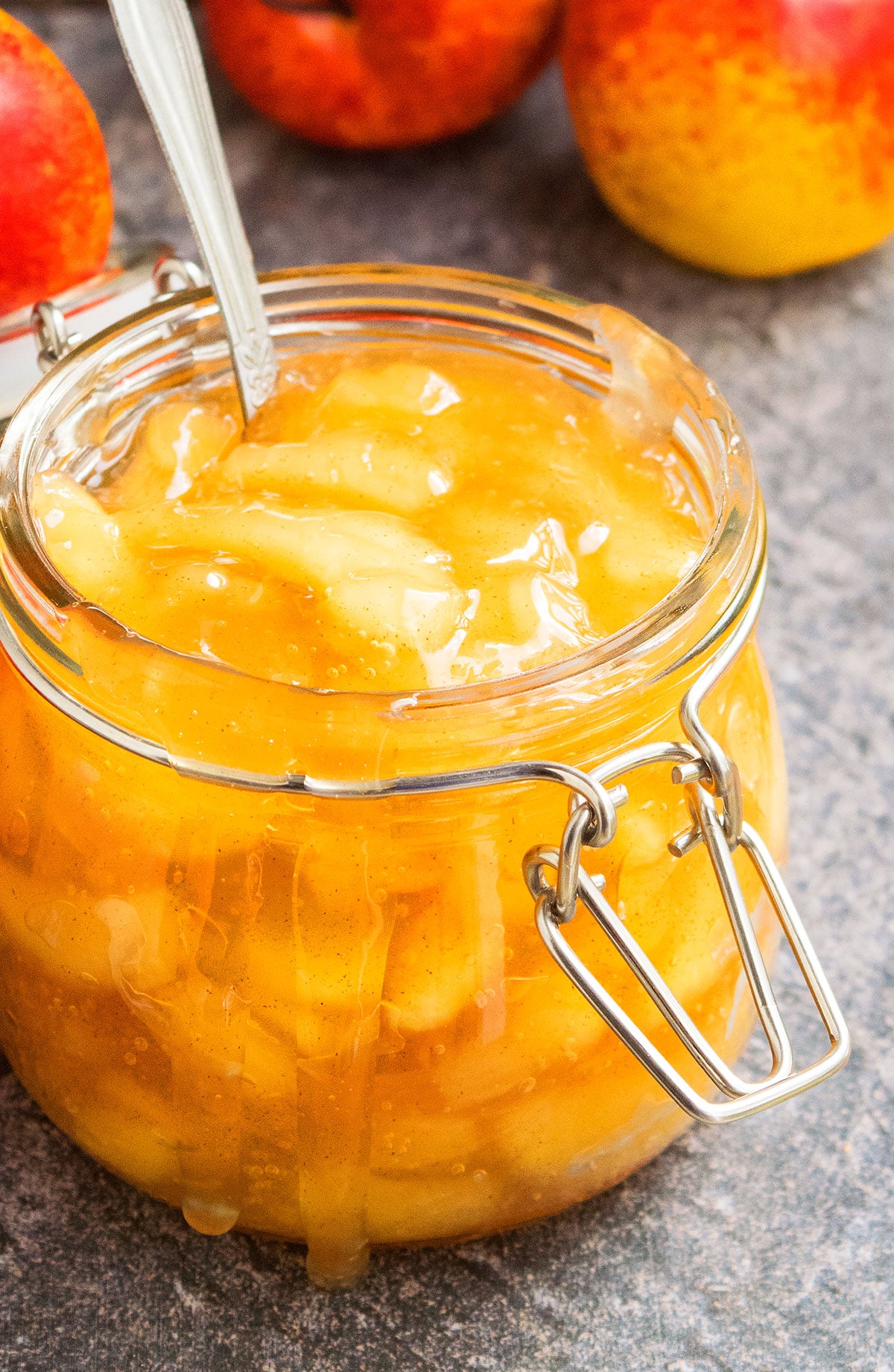The image features a glass container with a silver hinge and hardware, designed to lock its lid, which is currently open and pushed back. The container holds what appears to be homemade peach jam or preserves, characterized by vibrant yellowish-orange sliced peaches submerged in a liquidy, peach-flavored sauce. Some of the sauce is visibly oozing and dripping over the side of the container, indicating a luscious, overflowing texture. A metal spoon is placed inside the container. Behind the glass jar, there are three whole peaches. This setup rests on a gray table with a mixed dark and light gray textured surface, either a countertop or a textured gray placemat.